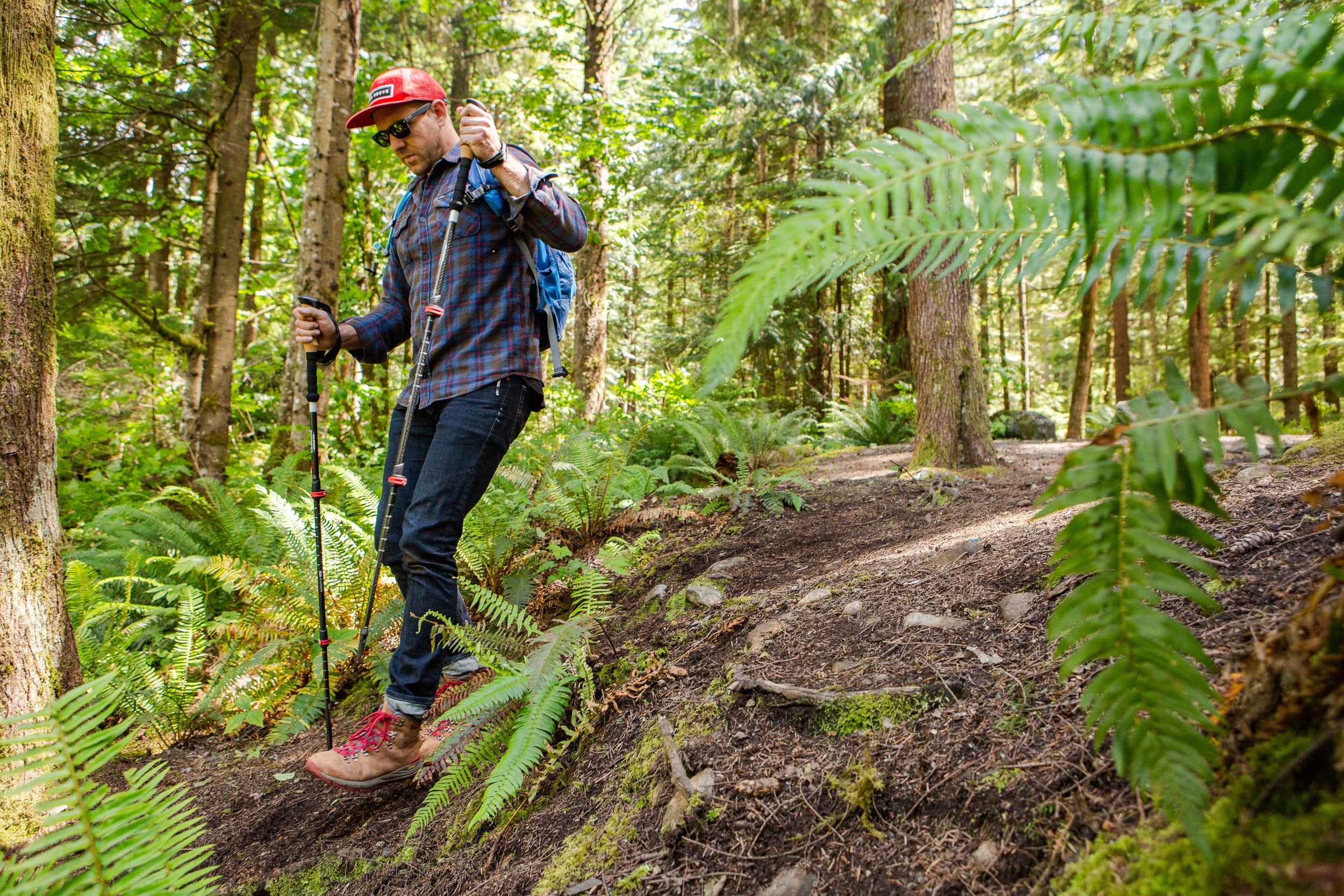The image is a detailed, horizontal landscape-oriented photograph, capturing a man navigating a steep, dirt slope in a heavily wooded forest. The hiker, dressed in blue jeans, a light-colored, dark blue plaid shirt, and brown hiking boots with red shoelaces, is stepping carefully down the hill, mindful of loose stones and the challenging terrain. He is equipped with a small blue backpack and uses a hiking staff in each hand to steady himself. His outfit includes a red baseball cap and dark sunglasses, which shield his eyes as the sun filters through the dense green canopy above. The trail he descends is characterized by bare dirt and a mixture of large and small tree trunks, ferns, and assorted ground vegetation, capturing the essence of a young woodland area. The man is seen in profile with his left side facing the viewer, and the photograph reflects a realistic style, emphasizing the natural beauty and challenges of the hiking environment.